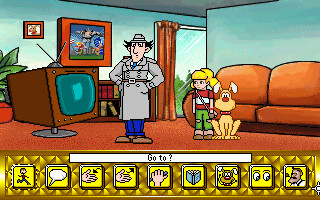The image is a screenshot from the Inspector Gadget video game. At the very bottom, there is a large yellow rectangle adorned with a diamond pattern. Within this yellow rectangle are nine smaller yellow squares, each containing a unique symbol. These symbols, from left to right, include: a person running, a speech bubble, a left hand with an arrow pointing inward, a left hand with an arrow pointing outward, a hand gripping a pen, an open blue book, a dog, a pair of eyes looking downward, and a man with a pipe in his mouth.

The upper right section of the image depicts a girl wearing a red shirt, white sleeves, green pants, and brown shoes, accompanied by a cartoon dog with a collar. They are positioned in front of a large leather couch against a blue wall. The background features a painting, a photo of a dog, and a window showcasing a view of a brown tree or possibly a TV screen. Standing in the center is Inspector Gadget himself, dressed in his iconic gray coat and hat, blue pants, and brown shoes.